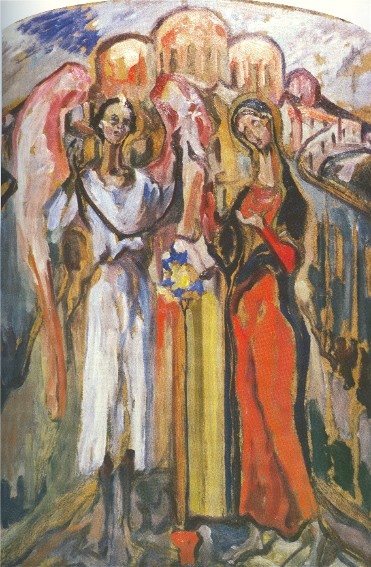The painting depicts two prominently featured humanoid figures standing in front of a yellowish, rectangular structure with a top that curves like the upper half of a circle. The front of this structure is a yellowish hue, transitioning to an orangey-brown on the left side. To the left stands a figure with an elongated neck, small head, dark skin, and black hair with a central white streak. This figure, dressed in a white robe tied with a black waist belt and armored shoes, also has red wings with white centers, resembling an angel. Their arms are stretched to the sides and raised. To the right, a woman with a distorted, wavering rectangular form wears an orange dress under a black robe that covers her head. Her face looks downwards. The background features a city or large building on a hill, characterized by light-colored structures and possibly bridge-like forms with pillars. The overall style is distorted, with the figures and background showing a blend of surreal elements and vivid colors.